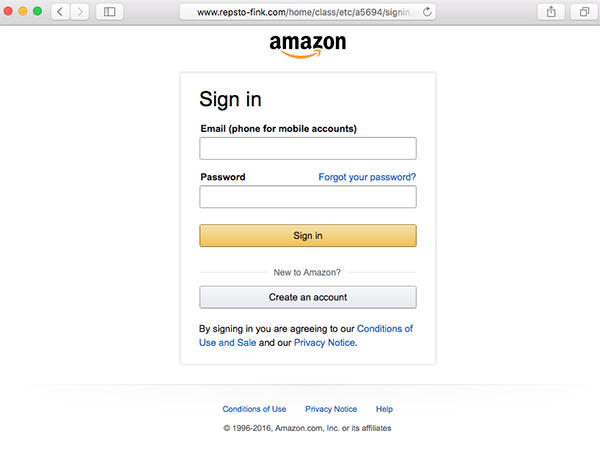The image depicts an open web browser window displaying the login page of Amazon's website. The URL at the top reads "www.reptsofink.com/home/class/etc." Beneath this, Amazon's logo is prominently featured in its traditional black lettering with a gold arrow pointing from left to right.

Central to the image is a vertical rectangle containing the sign-in interface. At the top, "Sign-In" is boldly written in black text. Below, there's a prompt to enter either an email or a mobile phone number, with corresponding input fields. Further down, a section to input the password is presented—above which, in blue text, is a "Forgot your password?" link for users who need to reset their credentials.

At the bottom of the form, a large gold bar labeled "Sign-In" awaits user interaction. Accompanying this is a message for new users: "New to Amazon?" followed by a link to create a new account. It also notes that by signing in, users agree to Amazon’s Conditions of Use and Sale, as well as its Privacy Notice. Additional clickable links for "Conditions of Use," "Privacy Notice," and "Help," along with the page's copyright information, are located at the very bottom.